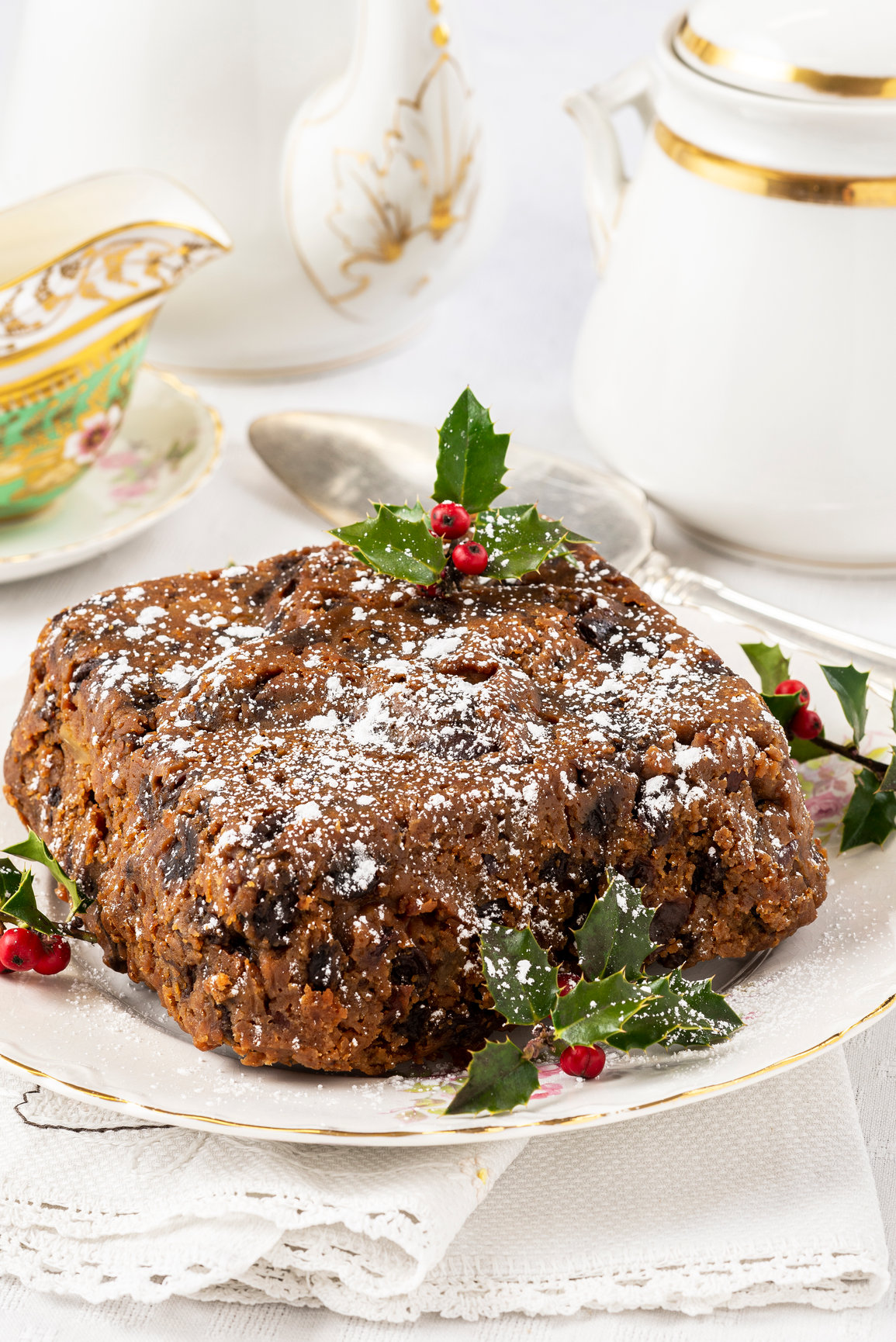This photograph captures a delectable holiday dessert displayed on a pristine, gilded white plate with a slender gold border. The centerpiece is a rectangular, cake-like brown loaf featuring chunks of a darker hue, possibly chocolate or preserved fruit, embedded within its sponge-like texture. The loaf is adorned with a festive garnish—clusters of red cranberries paired with vibrant green holly leaves. A whisper of powdered sugar is elegantly dusted atop the loaf, enhancing its holiday appeal. The dessert is set against a backdrop of a crisp white tablecloth, complemented by white decorative napkins beneath the plate. The background showcases a refined tea setting, complete with a gold-gilded tea kettle, white and gold china, and a serving spoon, adding an extra touch of elegance and festivity to the scene. This image, reminiscent of a recipe page from a gourmet cookbook, perfectly captures the essence of a charming holiday treat.